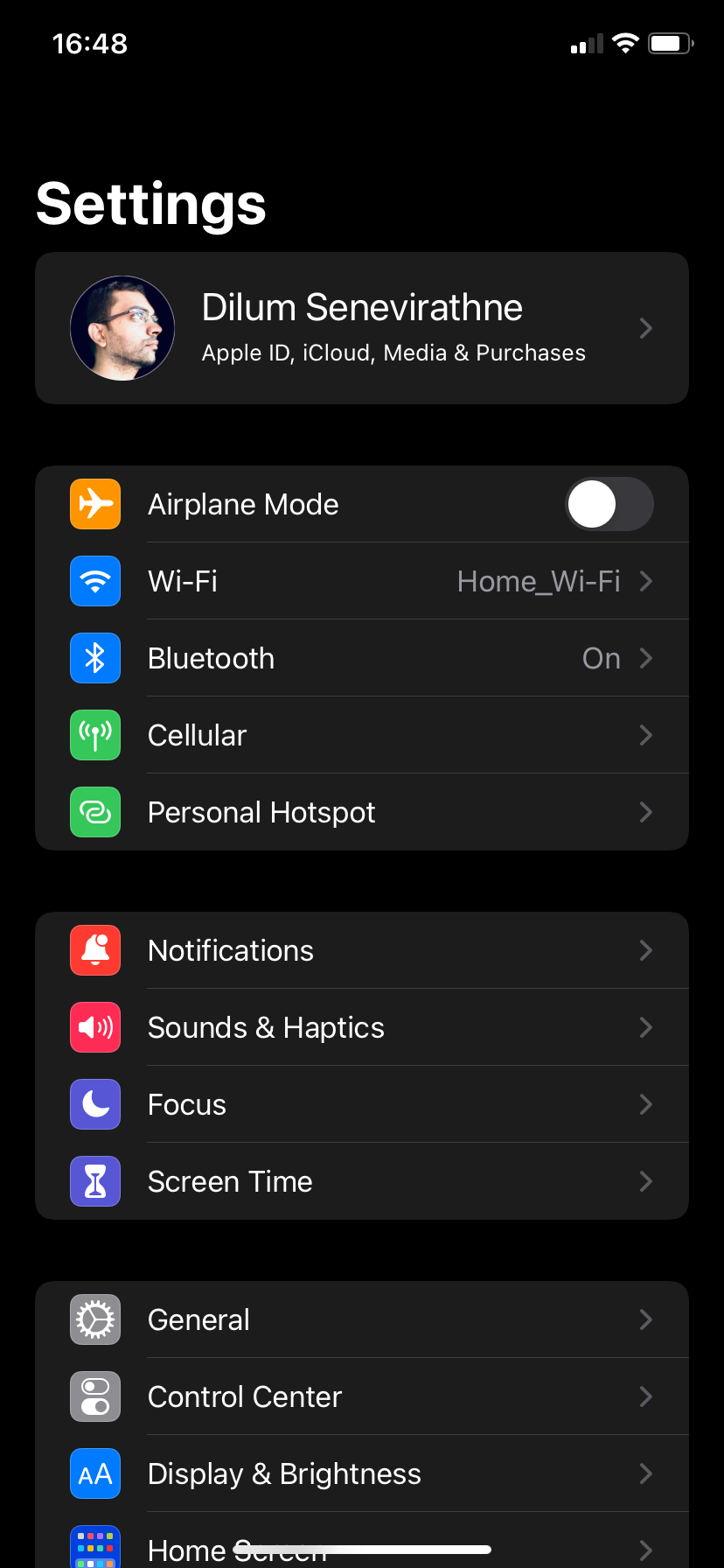This is a detailed screenshot of a cell phone displaying the "Settings" menu. At the top left, the time is shown as 16:48. On the top right, icons for cell phone signal, WiFi, and battery status are visible. Directly beneath these icons, "Settings" is prominently displayed in large, bold text. Below this, there is a dark grey, almost black, box featuring a circular profile picture to the left and the name "DILOM SENEVIRATNE" in prominent letters. Under the name, it mentions "Apple ID, iCloud, Media and Purchases."

Three additional dark grey boxes, similar in color to the profile box, are aligned vertically below. The first box includes options for Airplane Mode, WiFi, Bluetooth, Cellular, and Personal Hotspot. The second box lists settings for Notifications, Sound & Haptics, Focus, and Screen Time. The third box offers settings for General, Control Center, Display & Brightness, and Home Screen.

The background of the screen is black, though the outlined boxes are still distinctly visible. At the very bottom of the screen, just above the edge, there is a thin white line.